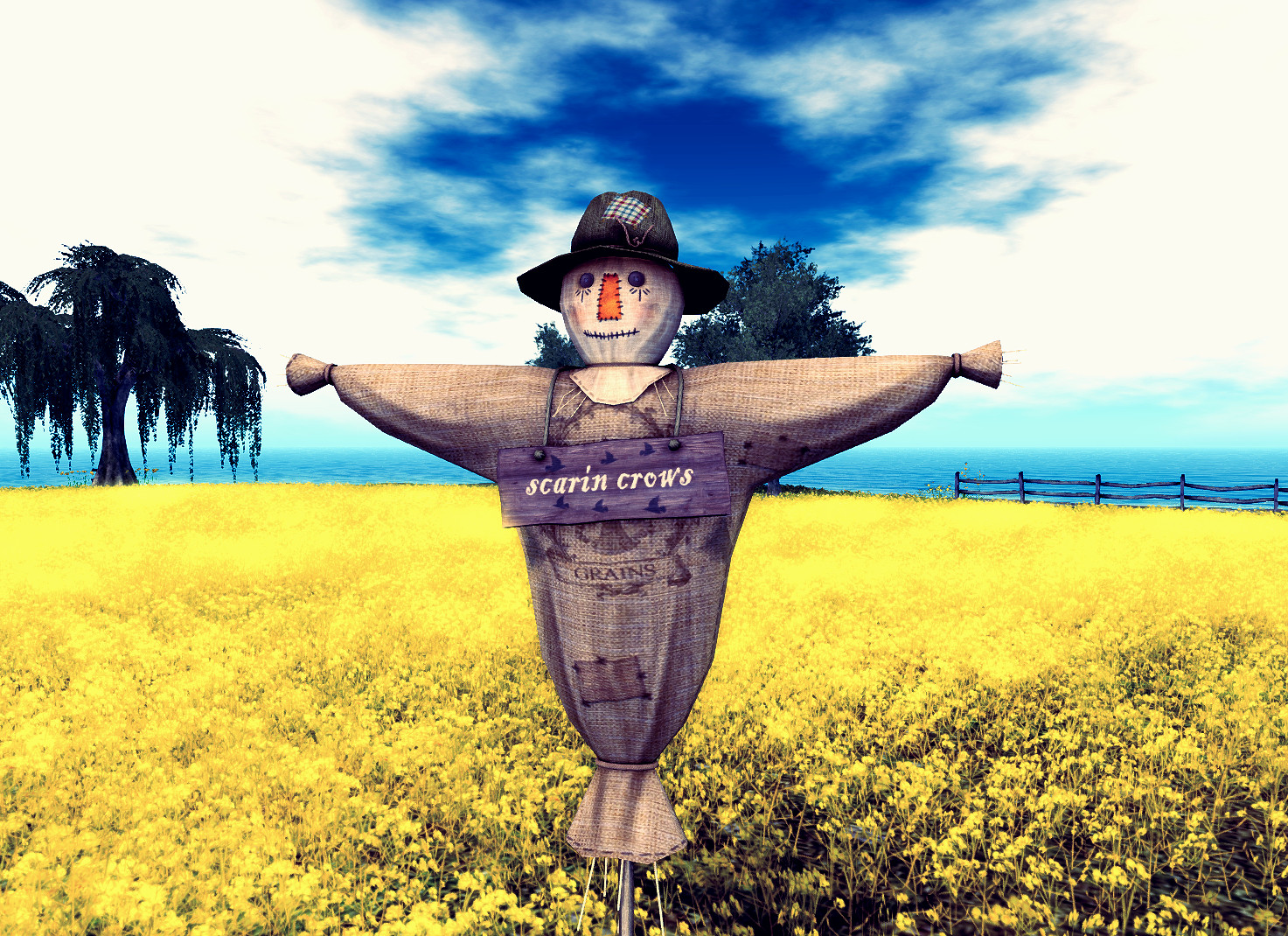This digitally-created image depicts a central scarecrow standing in an expansive field of striking yellow flowers, densely covering the ground beneath a vividly blue sky scattered with clouds. The field is part of a farm-like setting enveloping the scarecrow, which is notably attached to a metal rod and lacks typical appendages, coming to a tied bottom instead of legs. Adorned with a green sack and a black hat bearing a patch, the scarecrow wears a sign around its neck that reads "scaring crows" in white text. In the left background, a large, seemingly computer-generated weeping willow tree adds to the surreal quality of the scene, accompanied by two additional trees and an ocean backdrop complemented by an artificial lighting effect, suggesting a daytime ambiance. This crafted image bears the aesthetic hallmark of video game graphics, emphasizing its artificial and fantastical elements.